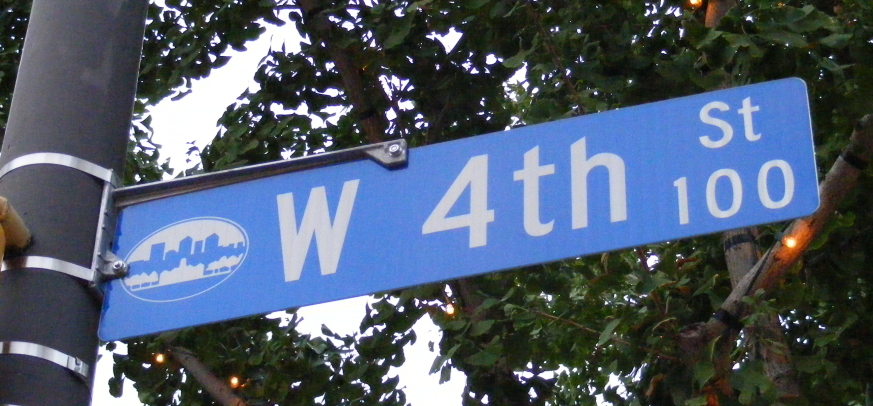In this detailed photograph, the focal point is a blue rectangular street sign mounted on a tall, black pole with silver accents, positioned on the left side of the image. The sign clearly displays "West 4th Street" in bold white font, accompanied by "100" in a slightly smaller font on the right, indicating the block number. To the left of the text, the sign features a city logo depicting a silhouette of tall buildings, adding a distinctive character to the image. Just barely visible is a finger pointing at the sign, adding a human element. The background on the right side captures medium-sized green leaves of several trees, one of which has an odd light among the foliage. The scene is set against a cloudy, overcast sky, contributing to an almost muted ambiance overall.